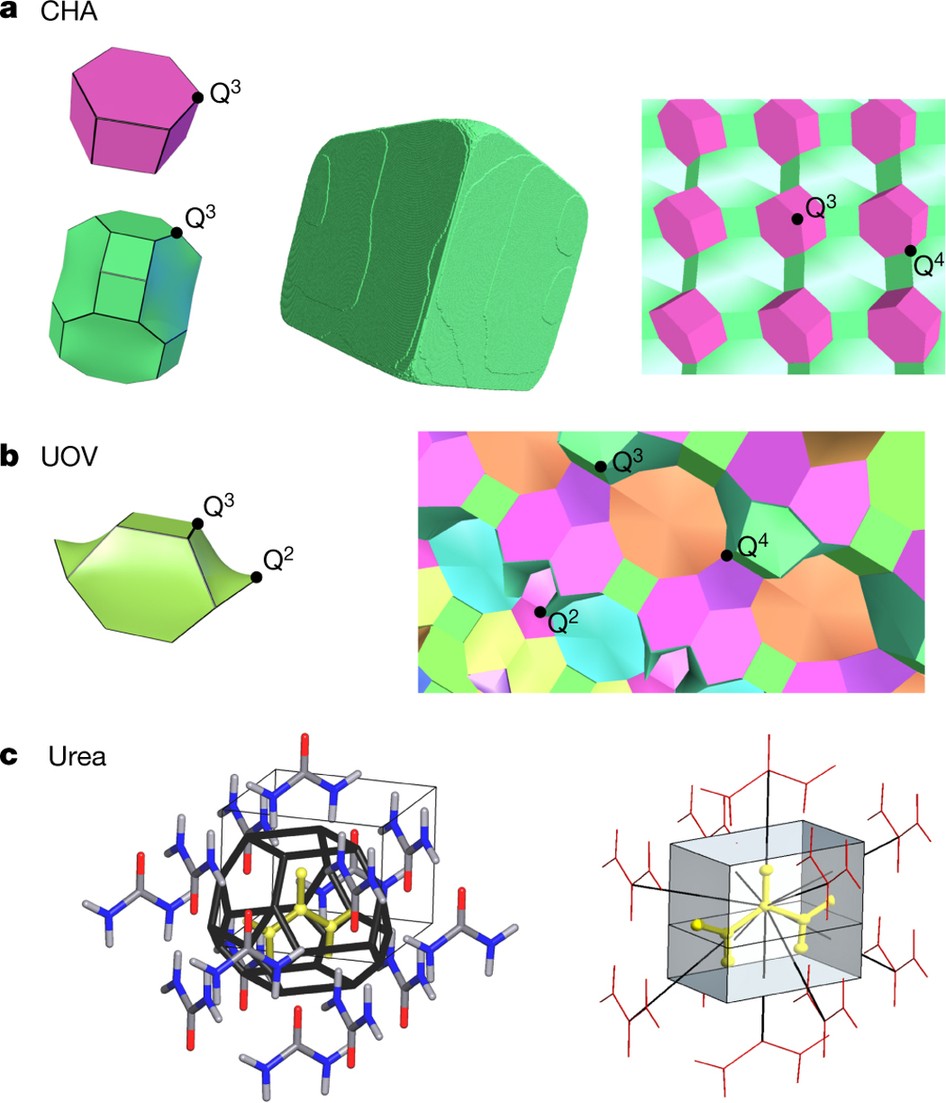The image features a detailed scientific infographic against a white background, showcasing molecules labeled A, B, and C. Under label A, there is a six-sided molecule labeled "CHI," accompanied by a 3D version labeled "Q3." Label B displays a molecule named "UOV" with intricate fins attached to a six-sided shape. Label C shows the complex structure of urea, characterized by numerous blue, red, and gray molecules arranged around a geometric circle and connected in a line framework. The right side of the image contrasts two structures of urea: the left one appears more complex and interconnected, while the right one has a more squarish, woven appearance. The infographic is vibrant, incorporating colors like green, pink, orange, blue, red, and yellow, and the design elements suggest computer-generated graphics with a medical emphasis. Additionally, there are floating pink geometric shapes on a green background, a green cube, rainbow-colored geometric patterns, and a grey rectangle with surrounding molecules depicted in the lower section.